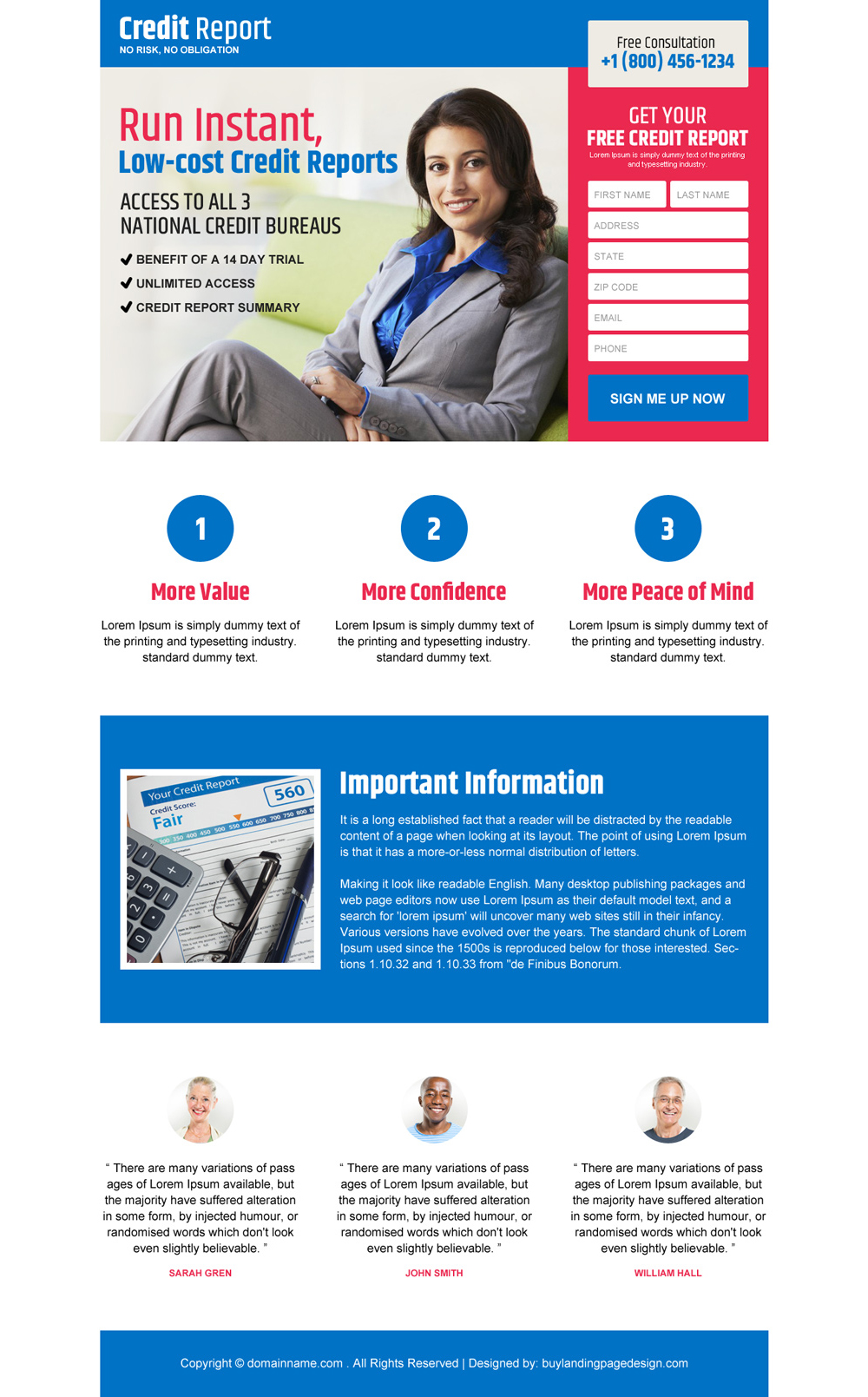The image features a digital advertisement with a dark blue header emblazoned with the words "Credit Report." Below the header, there is an image of a woman seated on a green sofa. She is dressed in a gray business suit with a blue collared shirt and has black hair cascading past her shoulders. She is posed with her legs crossed, exuding a professional demeanor.

In bold red letters across the image, the phrase "Run Instant" is prominently displayed, followed by the slogan "Low Cost Credit Reports" in blue. Underneath, various benefits of the service are listed in black text: "Access to all three national credit bureaus," "Benefit of a 14-day trial," "Unlimited access," and "Current report summary."

To the right side of the advertisement, there is a red call-to-action box that urges users to "Get Your Free Credit Report." Below it, there are several input fields for users to enter their personal information, accompanied by a blue button labeled "Sign Me Up Now."

At the bottom of the image, three blue circles are numbered one, two, and three. Each circle is followed by a benefit in red text: "More Value," "More Confidence," and "More Peace of Mind," respectively.